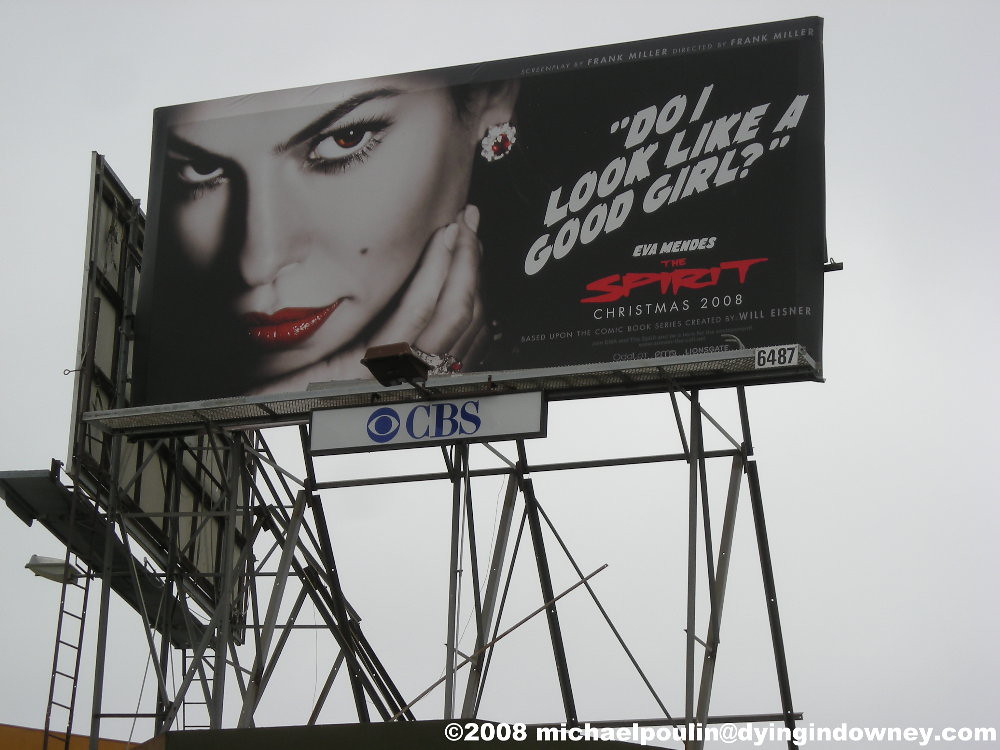This photograph showcases a billboard featuring a monochrome promo for the film "The Spirit." Dominating the center of the billboard is a vintage horror movie-style white font with the phrase, "Do I look like a good girl?" written in bold all-caps and surrounded by double quotation marks. Directly below, the actress's name, "Eva Mendes," appears, followed by the movie title "The Spirit" in a bold red font. The tagline at the bottom reads "Christmas 2008" in white font, signaling its release date. It also notes that the film is "Based upon the comic book series created by Will Eisner."

Prominently placed on the left side of the billboard is a striking image of Eva Mendes. The photograph is primarily black and white, but her lips are colored in a vivid red lipstick. Her irises are similarly tinted red, and she sports earrings featuring a central ruby stone. In the top right corner of the billboard, white text credits Frank Miller as both the screenwriter and director. Lastly, a CBS logo is affixed to the lower portion of the billboard.